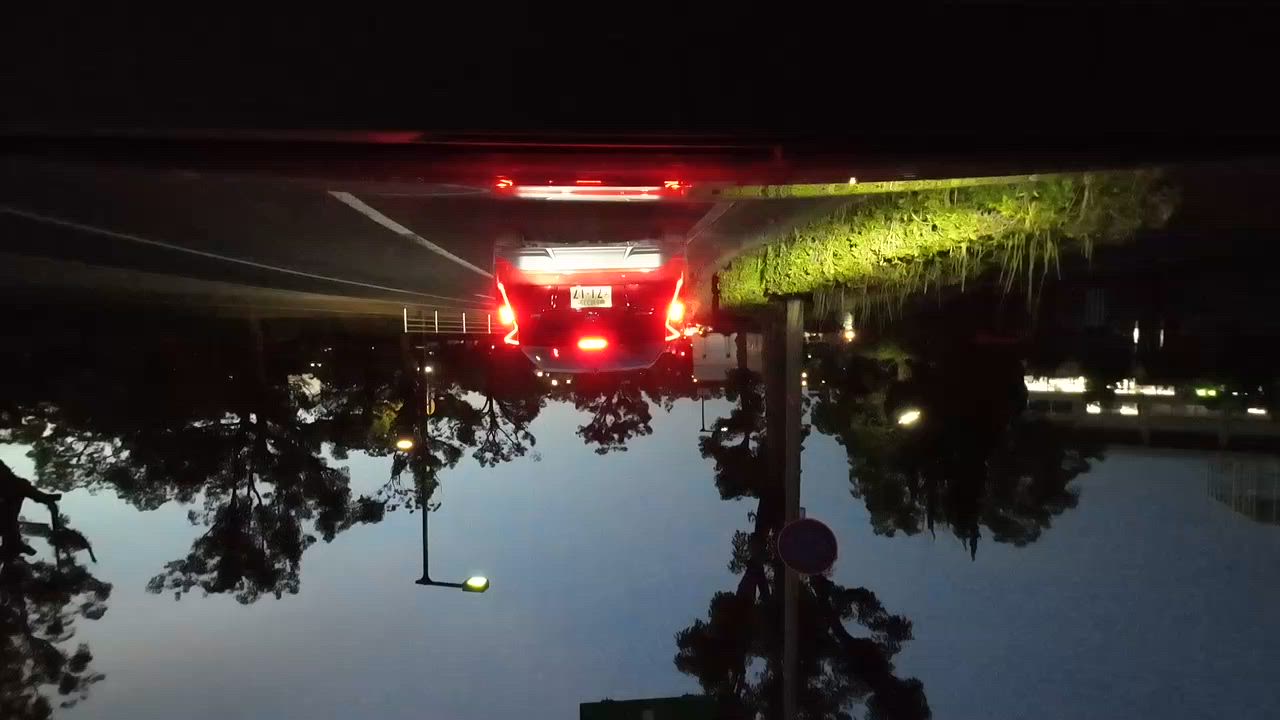The image depicts an inverted scene with an asphalt road running along the top. At the upper right corner, grassy hedges add a touch of greenery to the streetscape. A tree flanks either side of the frame, grounding the scene in nature. The bottom of the image resembles a darkened sky, hovering above which is a pole-mounted light, illuminating the area. The vivid red rear lights of a car punctuate the scene, adding brightness and depth. Another vehicle can be discerned, seemingly aligned with the grassy hedges, providing additional context and layering to the composition. On the far right, the image captures lights from a building, suggestive of a large assembly or structure, while a fence or railing divides the various elements, adding structure and framing the urban setting.